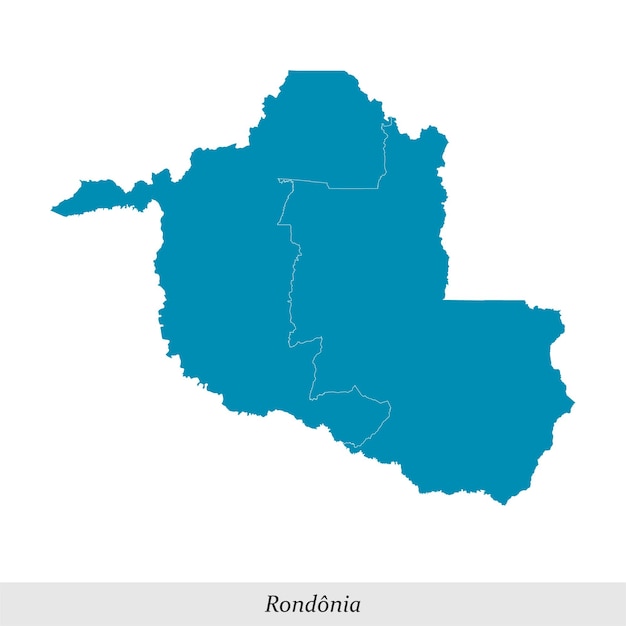This image features a map of a fictional place named Rondônia. The map is presented against a plain white background, and the area depicted is filled with a deep teal color. The shape of the region is somewhat oval, with a distinctive cut-out in the upper right corner and an additional protrusion in the upper left. A faint, squiggly white line, resembling a river or boundary, runs vertically through the center of the map. At the bottom of the image, there's a gray rectangular border containing the name "Rondônia" written in black text, with an accent over the "O".